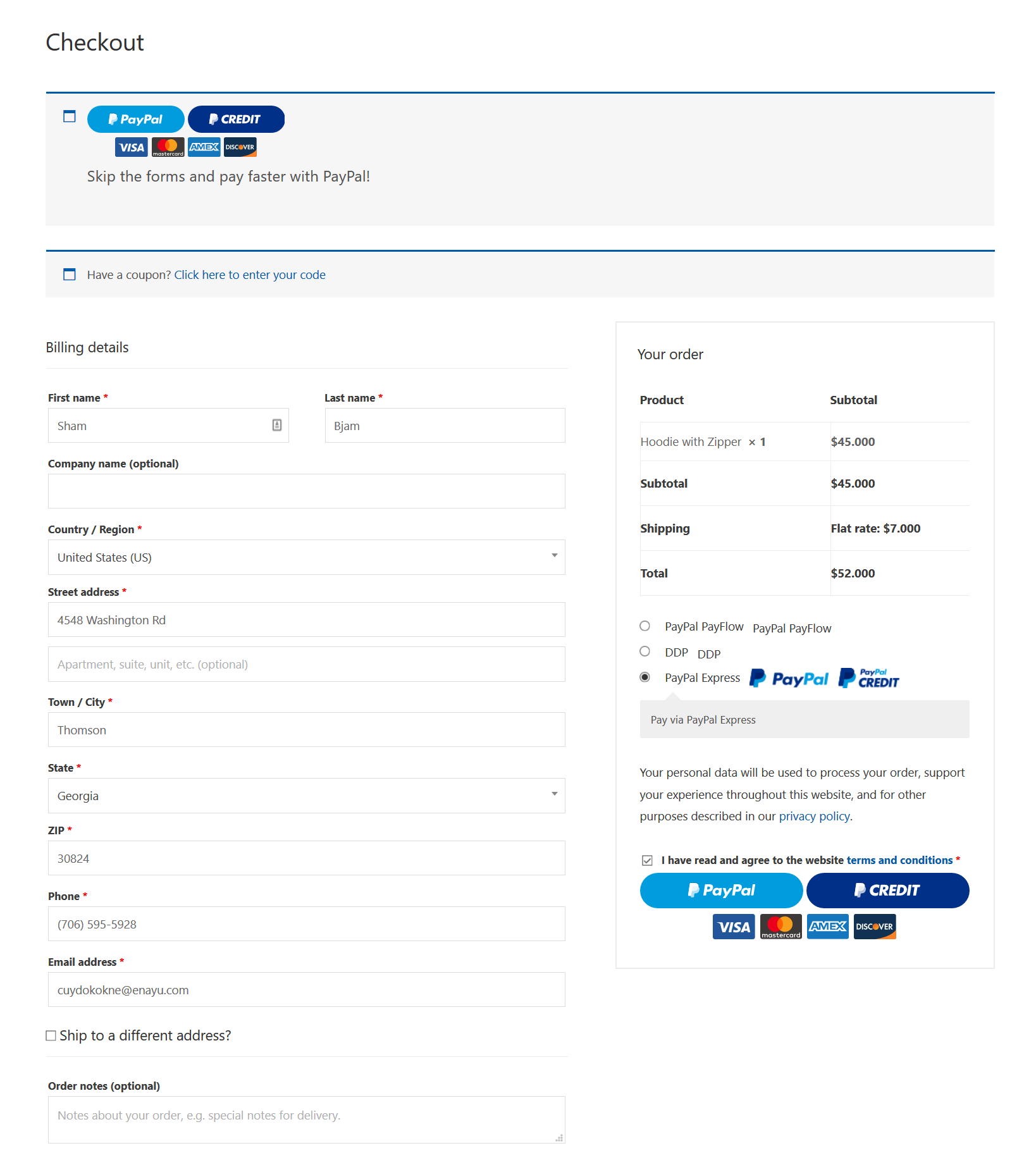This image depicts a detailed checkout page for an online purchase. The platform is unspecified, but it closely resembles a typical e-commerce site, possibly like Amazon. The checkout page allows the user to select their preferred payment method, such as PayPal or using a credit card. Credit card options include Visa, MasterCard, and Discover, among others. There is also an option to skip the card selection and directly proceed with PayPal.

Below the payment options, there's a checkbox for entering a coupon code that can be applied to the order. The billing details section is populated with the following information: 
- First Name: Sham (spelled S-H-A-M)
- Last Name: (possibly) Jam (spelled J-A-M)
- Country/Region: United States
- Street Address: 4548 Washington Road
- Town/City: Thomson
- State: Georgia
- ZIP Code: 30824

Additionally, a phone number and email address are included, though they are not shown in the transcription. There's also an option to ship the items to a different address if needed.

On the right side of the page, the order summary is displayed. The user is purchasing one "Hoodie with Zipper" priced at $45. The shipping fee is a flat rate of $7, bringing the total to $52. The chosen payment method for this transaction is PayPal.

Overall, the image provides a comprehensive view of the checkout process, billing information, and order summary for this online purchase.